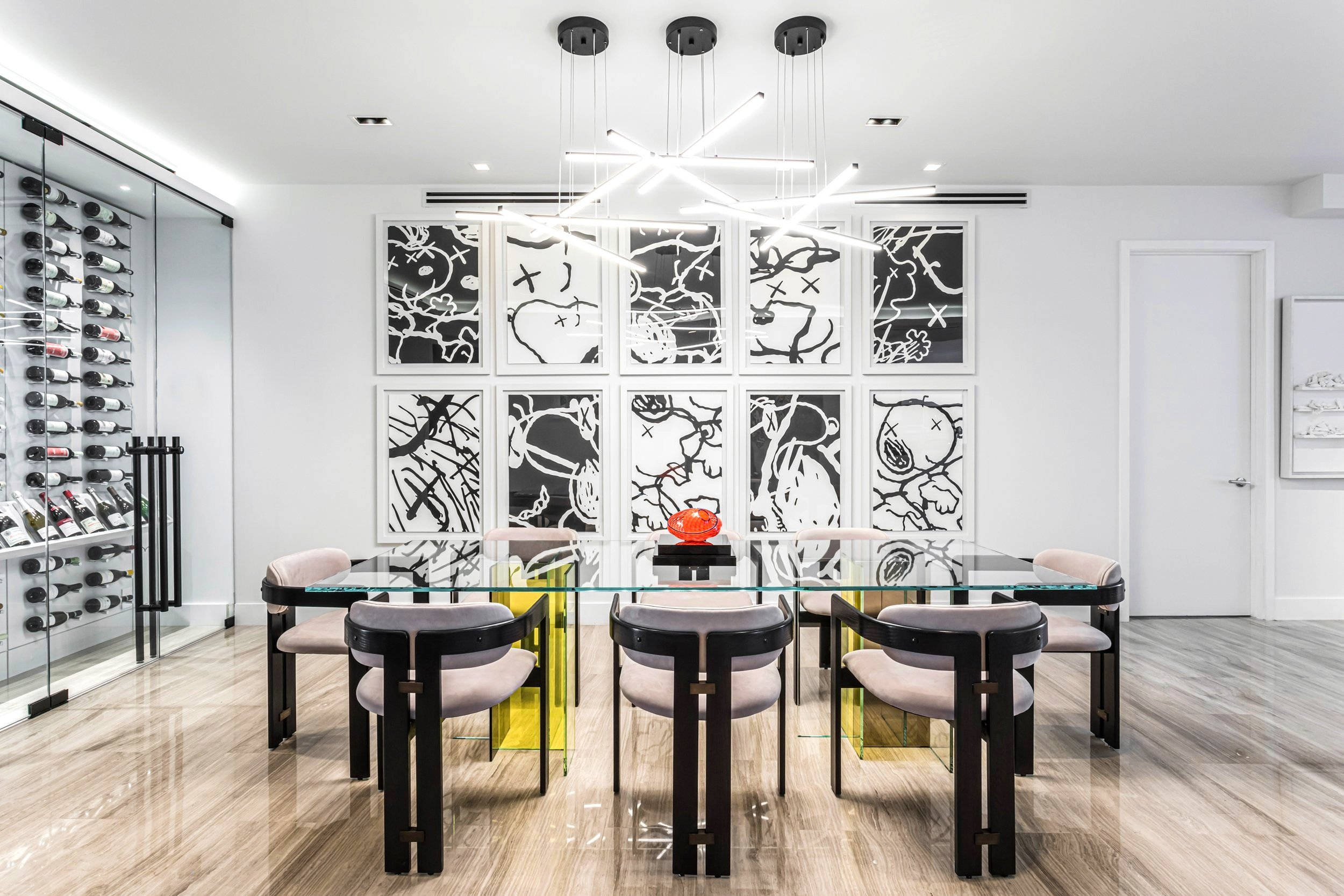This photo showcases a stylishly modern dining room with a clean, sophisticated aesthetic. At the center is a large glass dining table accented by unique black, square-shaped decor topped with a striking red glass orb. The table is supported by distinct yellow glass legs and is surrounded by eight high-backed chairs featuring black metal frames and gray cushions.

Above the table hangs an eye-catching chandelier with several elongated bars of light. The room's walls and ceiling are predominantly white, with a birch wood floor that reflects light brilliantly due to its high polish. To the left, there is a clearly visible wine collection, meticulously organized, with bottles displayed in a vertical fashion behind glass doors.

Behind the table is an intriguing collection of ten art prints depicting Snoopy from the Peanuts comic strip in various abstract, black-and-white poses. This pop art feels like a playful, unlicensed homage to the original character, adding an eclectic touch. Positioned subtly in the background is a yellow decoration that provides a burst of color amid the room's monochromatic palette and earth tones, enriching the modern art vibe. Overall, the space is impeccably designed, exuding a rich, high-end feel.